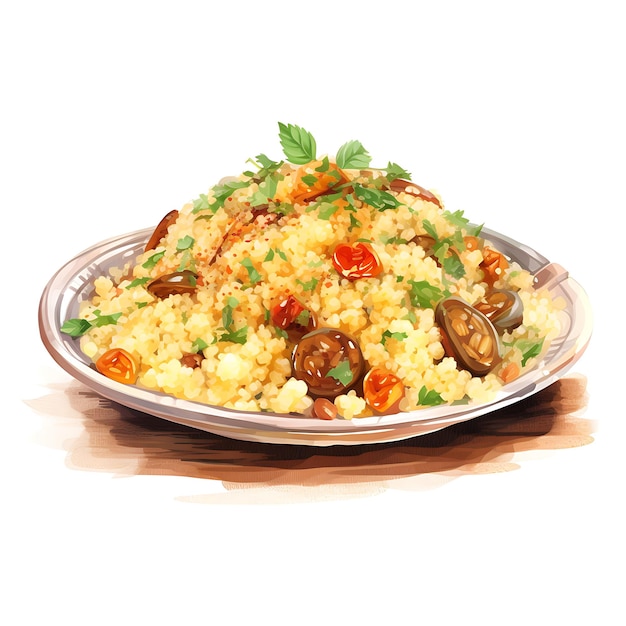The image depicts a detailed, computer-generated illustration of a single plate of food, primarily featuring a pile of white rice or rice cauliflower. The rice is generously coated with a creamy, yellow-tinted gravy. Scattered throughout the dish are chopped cherry tomatoes, jalapeno slices, and sprinkles of green herbs which resemble cilantro or parsley. Additionally, there are seasoned zucchini slices and peanuts integrated into the meal. The plate itself, exhibiting a curvature, is predominantly silver with an iridescent purplish tone on the left side, suggesting a high shine. This silver plate rests on a painted brown surface, providing the illusion of depth with a shadow underneath, indicating it was designed to appear three-dimensional. The composition has a polished advertisement-like quality, with no real paint involved.